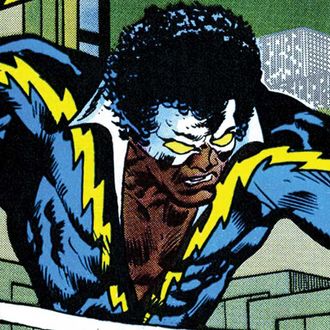This detailed cartoon image depicts an African American superhero set against a green sky and a cityscape with various skyscrapers in the background. He has curly black hair and is wearing a distinct white mask covering the top half of his face, revealing yellow eyes. His expression is a grunting grimace, and he is looking off to the side with a furrowed brow. 

The superhero's outfit is intricate, with a dark blue bodysuit featuring black accents. The suit is notably tight, vividly outlining his muscular physique. A striking feature of the costume is the deep V-neck that extends down the center of his chest, framed by a yellow lightning bolt pattern reaching up the sleeves. This V-neck reveals parts of his muscular torso. In front of the superhero, three crates can be seen, adding depth to the cityscape scene which includes a gray high-rise with white window details and a contrasting skyscraper in black and white with glass windows. The image is a vibrant, colorised comic book panel, possibly digital art, and embodies a dynamic superhero aesthetic without containing any textual elements.